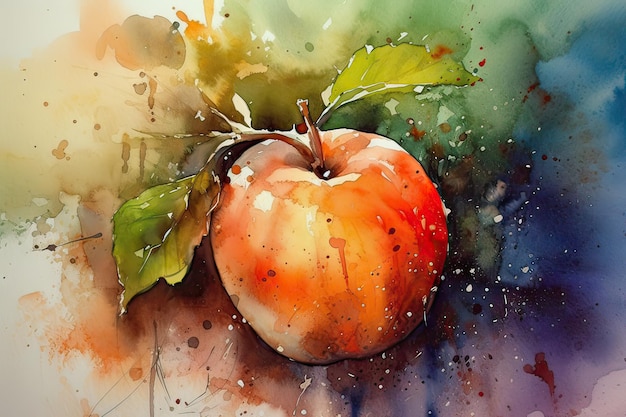This art piece is a vibrant watercolor painting depicting an apple set slightly off-center towards the right and somewhat down from the middle. The apple features a black outline with a wooden brown stem and two to three green leaves sprouting on either side. Its surface showcases a gradient from a darker red on the right to lighter, orangey-yellow hues on the left, with a creamy whitish center. The composition employs a blotchy, stylized technique, with splashes and dots of color decorating the apple and the surrounding space. The background transitions from neutral warm tones on the left, featuring whites, light oranges, and greens, to cooler tones on the right, including darker greens, blues, and purples. The entire piece creates a harmonious blend of colors, making the otherwise simple subject of the apple dynamic and eye-catching.